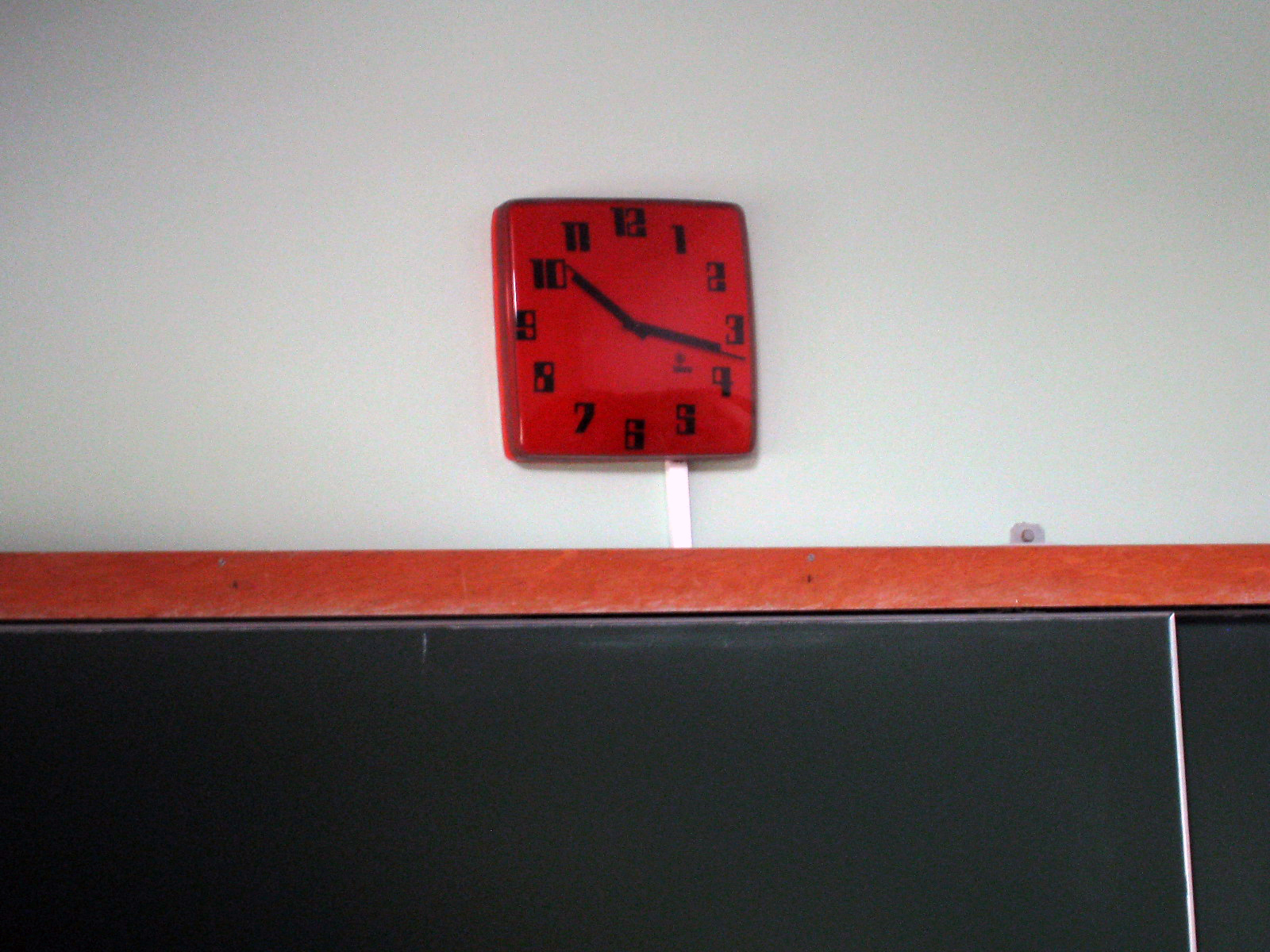This photograph captures an upward perspective of a classroom wall, prominently featuring a vintage, square-shaped wall clock at its center. The clock, striking with its red frame and sleek glass-like surface, showcases bold, blocky numerals reminiscent of the 1970s style. Its black hands, positioned at 3:50, stand out against the clock's minimalist face. Directly below the clock is a horizontal strip of reddish-brown wood framing, which likely serves as a shelf or trim. Beneath this wooden accent lies a large, greenish surface that appears to be a chalkboard, evocative of traditional classroom settings. The composition of the image highlights the timeless ambiance of an educational environment through its distinctive, retro elements.